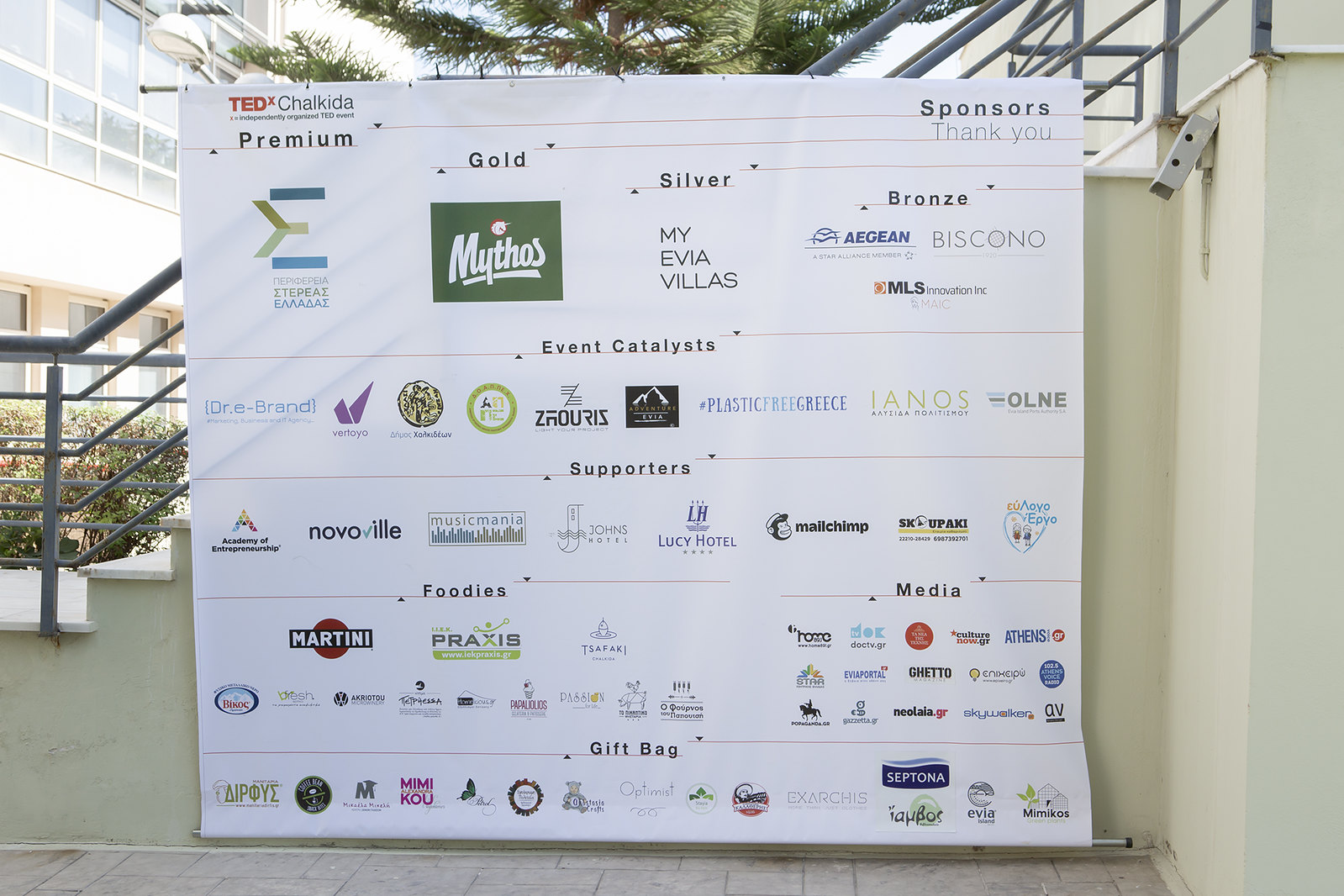The photograph, taken outdoors during the daytime, captures a large, square, white promotional backboard banner mounted on a set of light-colored concrete stairs with grey railings. The stairs lead upwards. The background includes a white building, blue sky, and a palm tree. The banner, which measures approximately six inches wide by four inches high in the photograph, showcases various business logos as a tribute to the event’s sponsors. 

In the upper left corner of the banner, the text "TEDxChalkida" is prominently displayed in red and black with the tagline "X = independently organized TED event" beneath it. The top right corner reads "Sponsors, Thank You" in two lines. The banner categorizes sponsors into Premium, Gold, Silver, and Bronze tiers and lists their names underneath each category. 

The Premium sponsor appears to have a Greek name. The Gold sponsor is Mythos, while the Silver sponsor is My Evia Vias. The Bronze sponsors include Aegean (a Star Alliance member), Piscano, and MLS Innovation, Inc. 

Below these tiers, additional categories labeled Event Catalysts, Supporters, Foodies, Media, and Gift Bags list various other sponsors. Notable mentions in these groups include the Academy of Entrepreneurship, Novoville, Martini, BeFresh, Praxis, Star, Propaganda, and numerous unreadable Greek brands.

The banner collectively honors around 50 sponsors, meticulously categorized and distributed across different levels of contribution, displaying the significant support for the independently organized TEDx event in Chalkida.